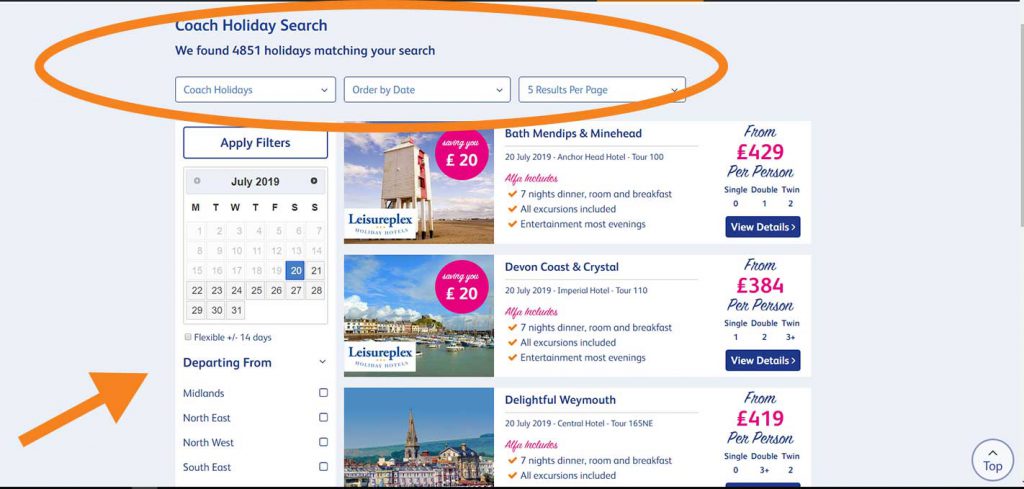The image is a screenshot of a travel website interface, focusing on coach holiday searches. At the top of the page, circled in orange, is the section labeled "Coach Holiday Search." Beneath this header, it indicates that there are 4,851 holidays matching the search criteria. Three white rectangles display options: "Coach Holidays," "Order by Date," and "Five Results per Page." 

Towards the center-left, there's a calendar showing July 2019, with the 20th highlighted in blue. Below the calendar, the text reads "Departing from," followed by multiple regions: Midlands, Northeast, Northwest, and Southeast, with a red arrow pointing to these departure options.

To the right, three images showcase different destinations. The first destination is labeled "Bath, Mendips, and Minehead," priced from 429 lira per person, highlighted in purple. The image of this location includes a feature of the LeisurePlex. The second destination listed is "Devon Coast and Crystal," from 348 lira per person, also priced in purple, accompanied by an image of another LeisurePlex in the area. The third destination, "Delightful Weymouth," is shown as costing from 449 lira per person, with the pricing in purple.

Each destination is accompanied by visual imagery to attract potential travelers, featuring scenic photographs that represent the locations.